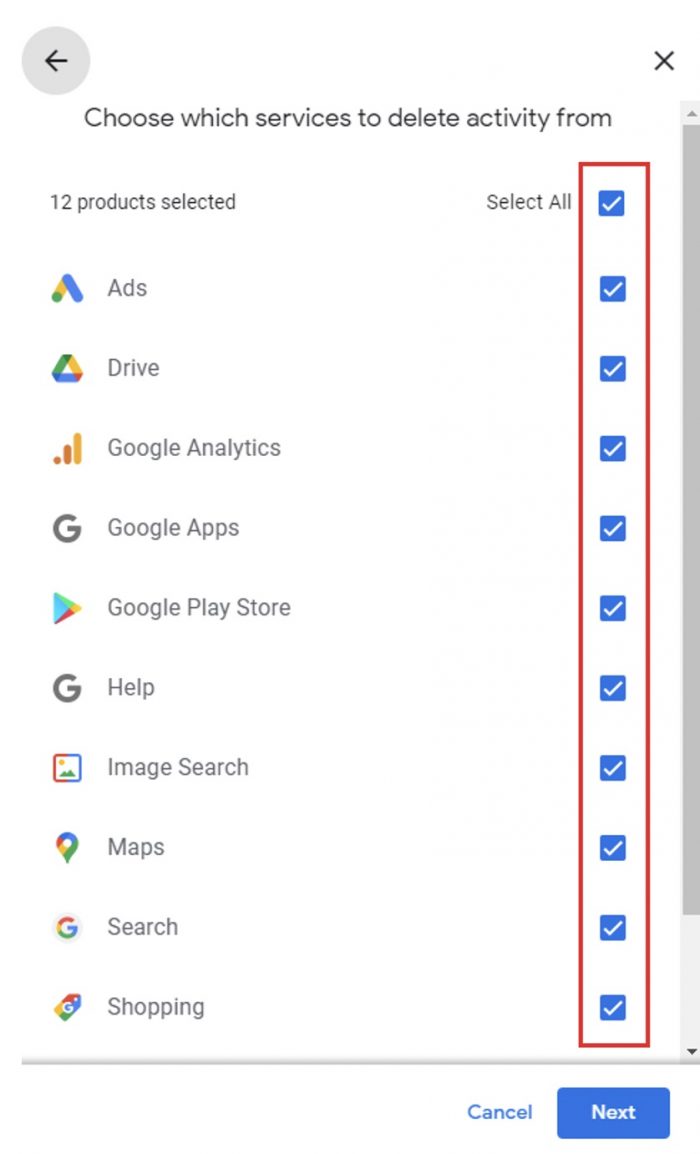At the top of the image, there is a gray circle followed by a left-facing arrow, indicating a back or previous action. Below this, an instruction reads, "Choose which services to detect by default," followed by a gray bar. The main section of the image displays a table with a red border that contains eleven squares, each numbered from 1 to 11. Inside the squares, there are blue backgrounds with white check marks. The squares are labeled with various Google services: Ads, Drive, Google Analytics, Google Apps, Google Play Store, Google Image Search, Maps, Google Search, and Shopping. The background of the image is predominantly white. Towards the bottom, there is a blue "Cancel" button and a "Next" button, both on a white background. The right side of the screen lists numbers from 1 to 10 consecutively.